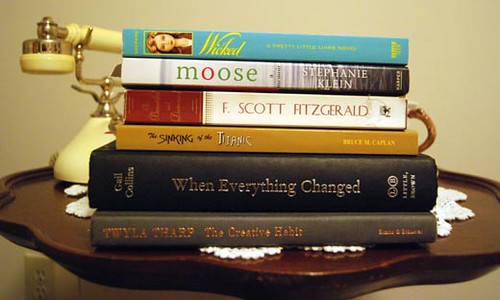In the photograph, there is a small, dark brown table adorned with a large, intricate doily. On top of the doily sits a stack of six books, their spines clearly visible. From top to bottom, the books are titled *Wicked*, *Moose*, an unidentified work by F. Scott Fitzgerald, *The Sinking of the Titanic*, *When Everything Changed*, and *The Creative Habit* by Twyla Tharp. Alongside the books rests an old-fashioned European handset telephone, reminiscent of the 1950s or 1960s, complete with an earpiece and mouthpiece. In the background, a tea kettle with a brown handle is just barely visible. The scene is set against a greenish wall, providing a nostalgic and vintage ambiance.